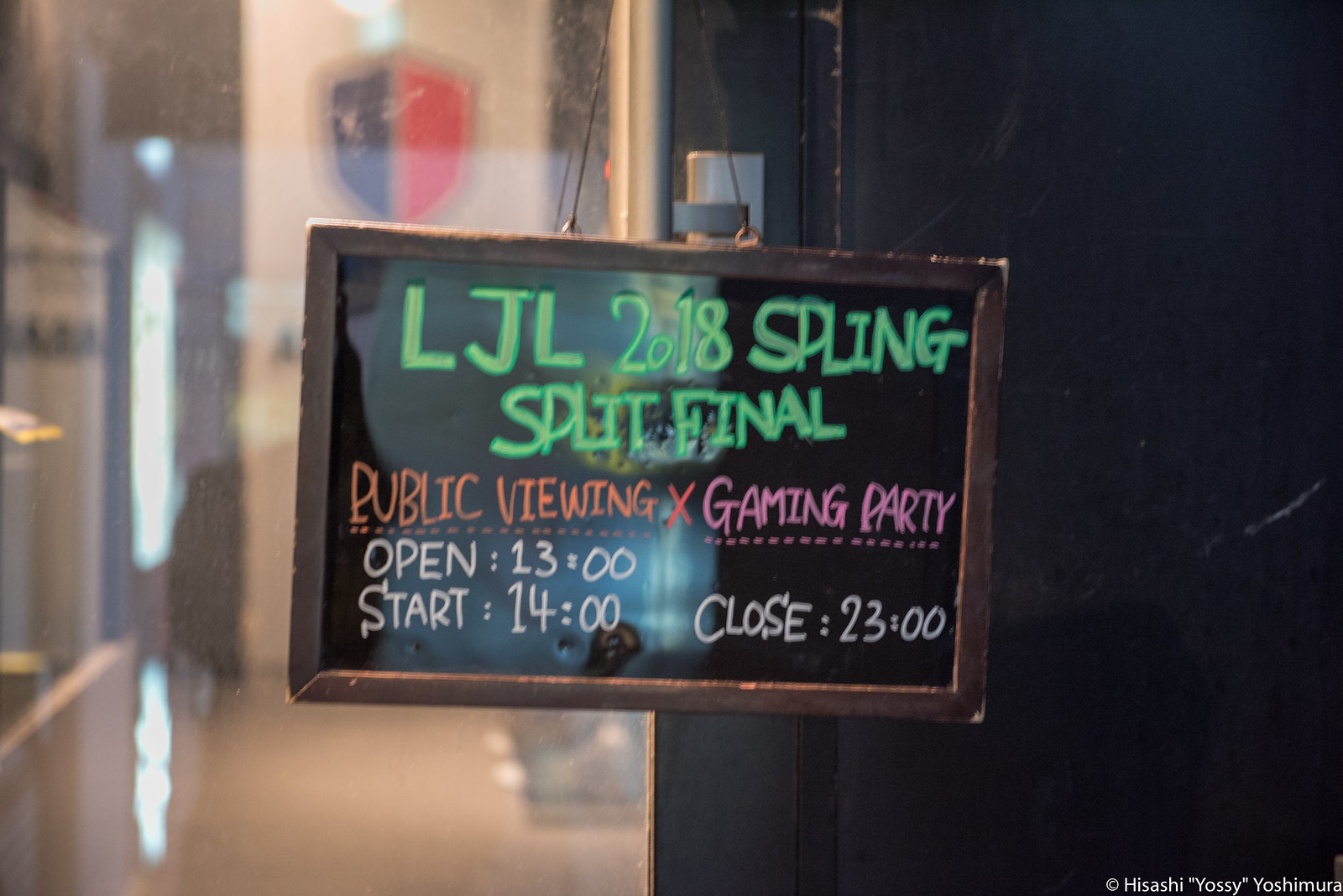This color photograph captures a store hour sign hanging in a shop window. The sign has a wooden frame and is suspended by strings. The top half of the sign, resembling a black chalkboard, features green text that reads "LJL 2018 Spring Split Final." Below that, in red text, it states "Public Viewing," followed by the schedule: "Open 13:00, Start 14:00, Close 23:00." To enhance the festive atmosphere, the words "Gaming Party" are highlighted in pink. Through the window, the left side of the store interior is dimly visible, revealing a decorative shield on the wall—its left half is black and the right half is red. The right side of the view through the window is predominantly black. In the lower right corner of the sign, small text reads, "© 2018 Yoshimura."